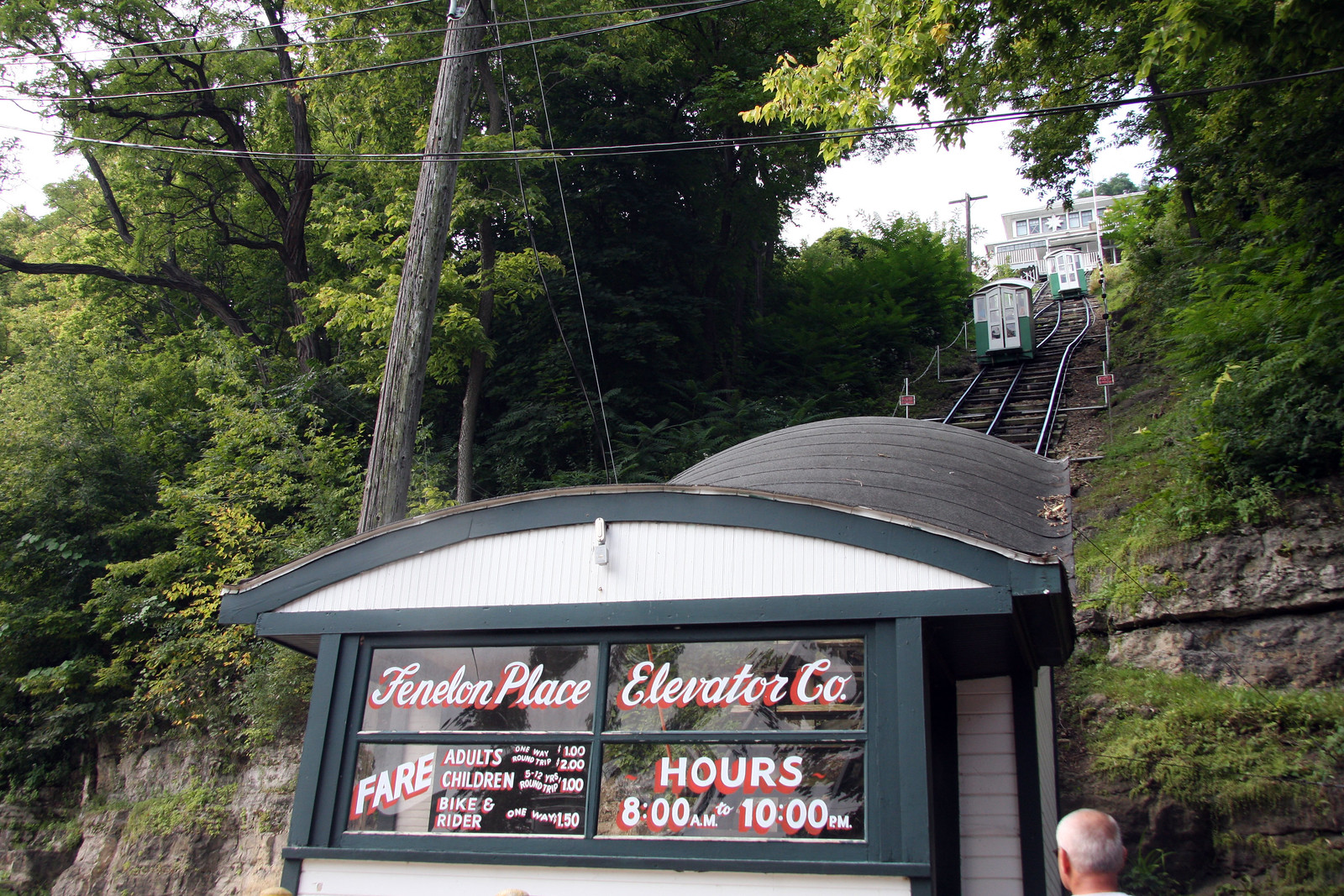The image depicts a hillside with a tram, labeled "Fenelon Place Elevator Company," ascending on tracks built into a rocky incline. Trees border both sides of the tracks, with dense foliage on the left and slightly sparser greenery on the right, partially overgrown with ivy or weeds. A prominent telephone pole with power lines stands to the left. In front of the tram, a covered entrance platform features dark silver, blue, and white elements. The tram's front window displays operating hours, "8 a.m. to 10 p.m.", and fare information for adults, children, and bike riders, written in white and pink shadowed text. A man with gray, balding hair is positioned in the lower right corner, appearing to engage with or observe the tram. The tracks extend to the top of the hill, where a white building against a white sky marks the endpoint of the journey.